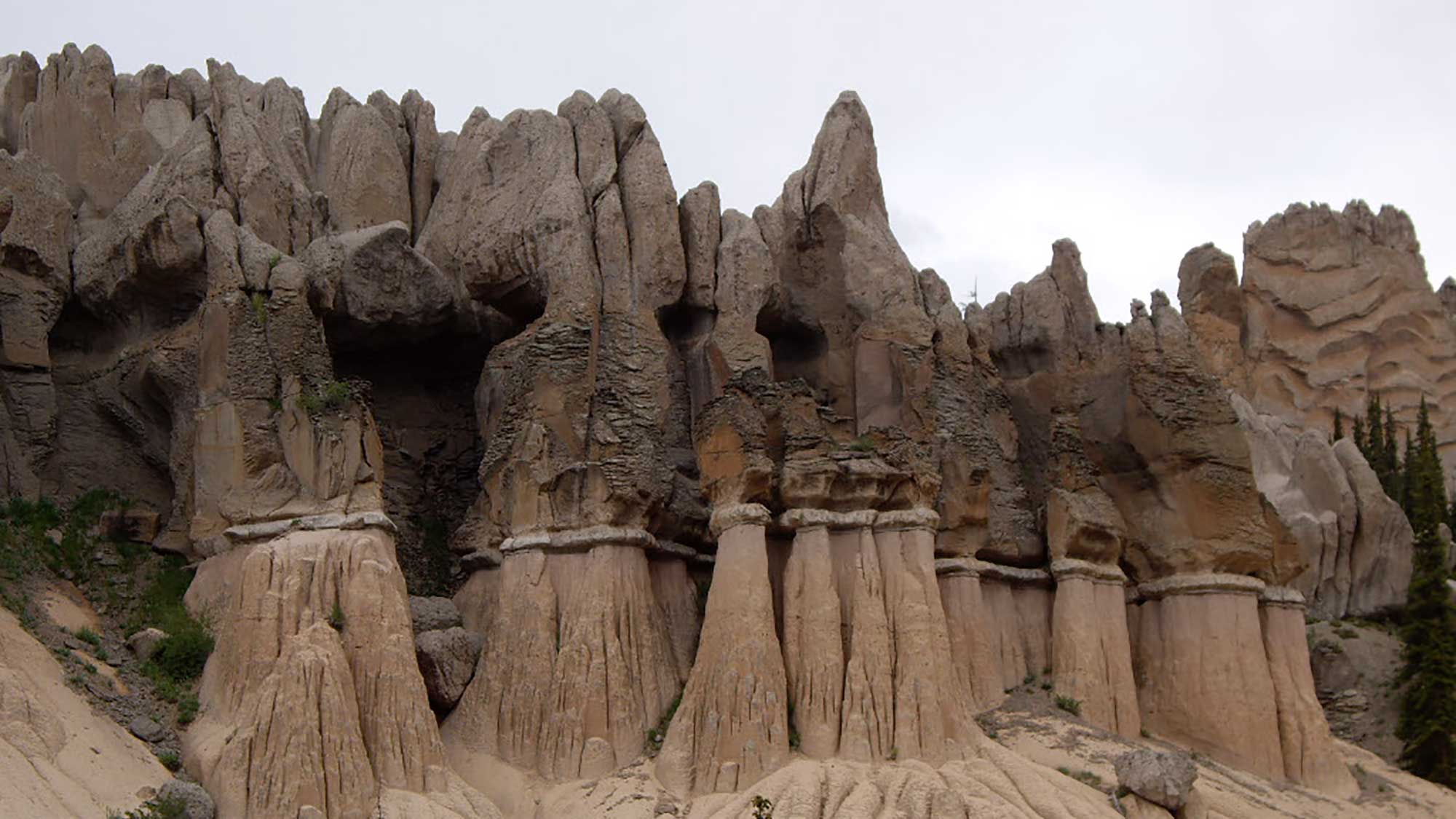The image captures a striking desert canyon landscape featuring a series of tall, cylindrical rock formations, possibly formed by both natural erosion and human intervention. The canyon walls showcase a distinct vein of rock that climbs up the cylinders, flares out, and blends back into the rugged, crunchy rock that makes up the rest of the terrain. The bottom of the scene is sandy and slopes outward, creating a natural pathway. To the right, there are pine trees adding a touch of greenery, while some grassy bushes grow on the left. The sky is a soft blue, suggesting a clear, bright day. The rock formations present a horizontally segmented, slightly pointed surface, resembling a complex and ancient natural marvel. The overall area appears to be a mountainous region with some greenery and gravel interspersed among the rocks, contributing to the majestic and cavernous feel of the scene.